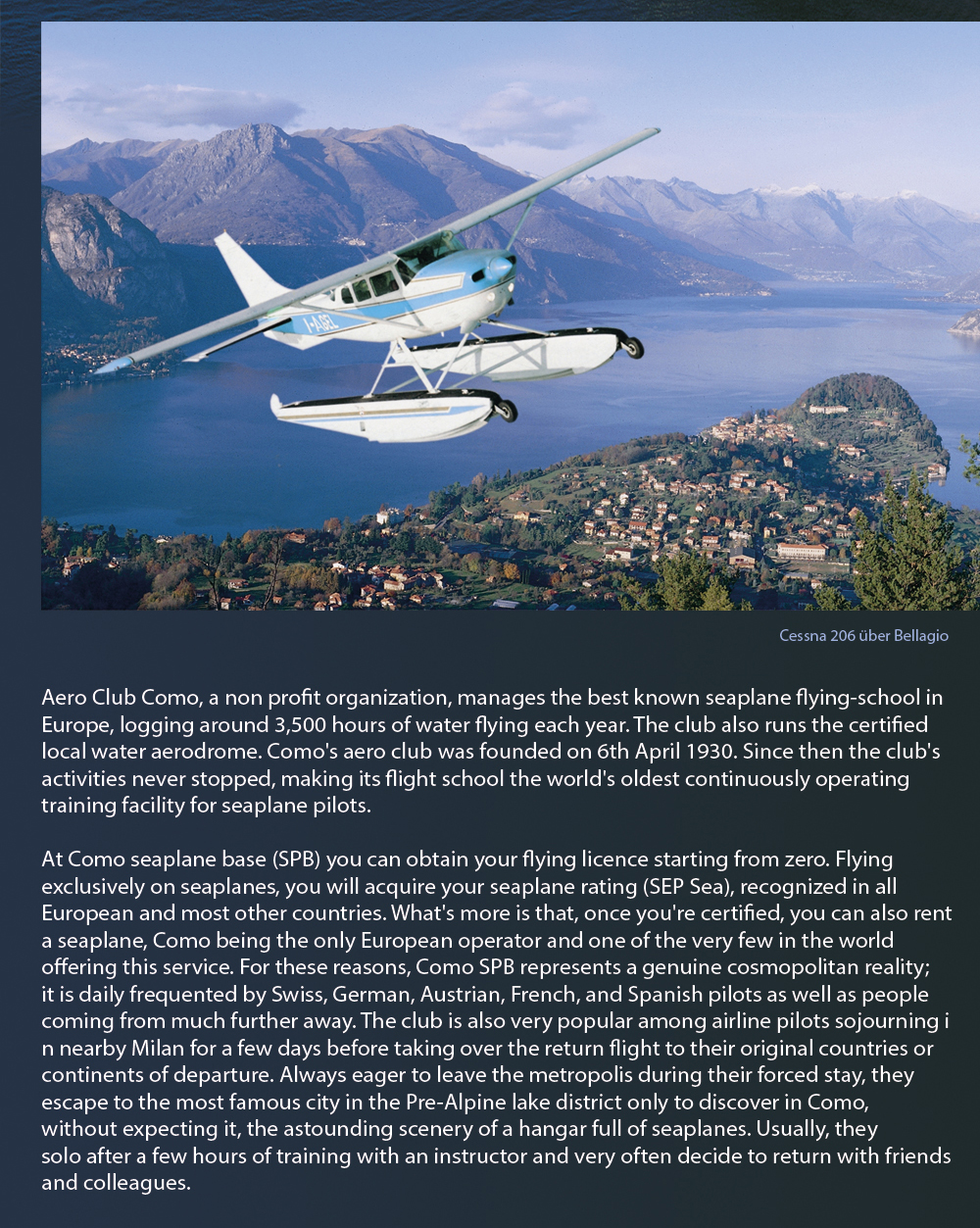This is a color photograph taken during the day of a blue and white seaplane, identified as a Cessna 206 Uber Bellagio, flying over a large body of water with a mountainous backdrop. The seaplane, equipped with pontoons, is flying to the right at an altitude of approximately 1,500 feet, towering above a small city with scattered homes on a land peninsula. The scene extends to feature substantial waterway views, possibly a large river, tributary, or an ocean inlet. Beneath the photograph, descriptive text highlights the Aero Club Como, a non-profit organization renowned for managing the best-known seaplane flying school in Europe. Founded on April 6, 1930, Como's Aero Club has maintained continuous operation, making it the oldest seaplane pilot training facility in the world. The club logs around 3,500 hours of water flying annually and operates a certified water aerodrome. Pilots can obtain flying licenses and seaplane ratings recognized across Europe and many other countries, with certified individuals gaining the option to rent a seaplane. This club is frequented by pilots from various regions including Switzerland, Germany, Austria, France, and Spain, as well as those from further afield, and is popular among airline pilots laying over in nearby Milan. The detailed text describes Como's compelling allure for aviators, highlighting its cosmopolitan nature and the breathtaking scenery, making it a unique destination for seaplane training and flights.